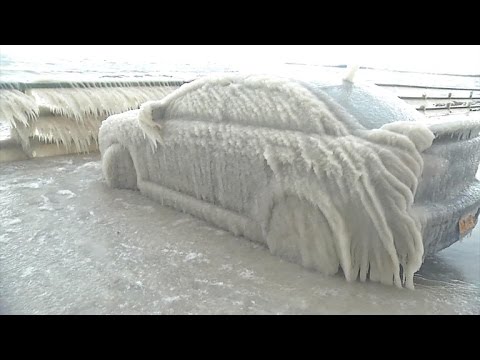This horizontally aligned rectangular photograph, framed by thick black borders on the top and bottom, captures a remarkable scene of an outdoor setting blanketed in ice. A sedan is prominently featured, with its entire left side, back end, and partially visible license plate—which is an orangish-yellow hue—encased in layers of brown, tan, and white ice. The vehicle appears to be frozen at an angle, with streaks of snow and ice clinging to its surface, suggesting it was battered by a powerful windblown storm. Icicles dangle from the rear bumper, and the front tires are aimed to the left, entrenched in the icy ground.

Accompanying the car is a pedestrian railing, similarly shrouded in ice that stands horizontally as if it froze mid-flight. The ground is entirely flat and covered in a mix of brown, tan, and white ice, further highlighting the aftermath of the storm. To the upper right of the image, a fence is partially visible, while in the background, layers of long icicles cascade from what looks like a small waterfall. Beyond this icy barrier, a body of water can be seen with dark waves rolling against the backdrop of a white sky. This chilling yet captivating scene illustrates the sheer power and beauty of nature's icy grip.